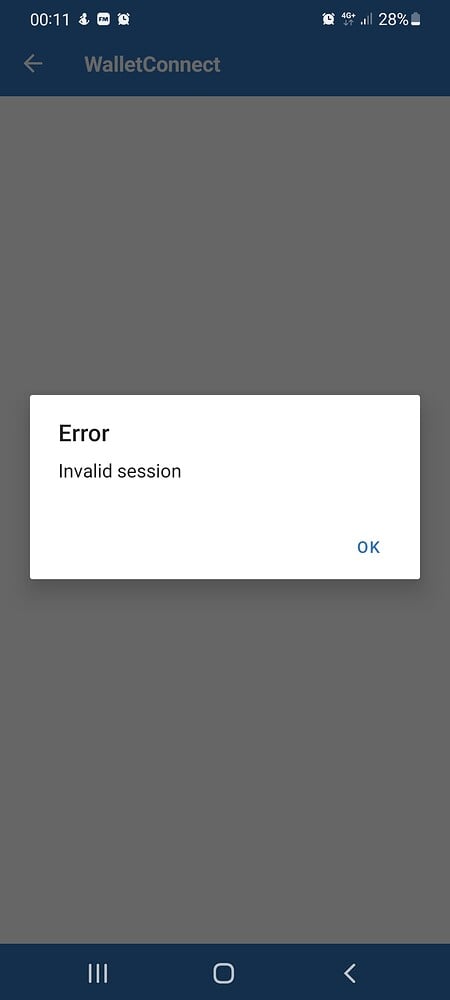This detailed 4K screenshot captures an interface from the Wallet Connect website. At the very top, there's a gray navigation bar containing a left-facing arrow and the words "WalletConnect" merged into a single term. Below this navigation bar lies the main body of the web page, which is predominantly gray in color.

Overlaying the gray background is a prominent white dialog box featuring an error message in black text that reads "Error: Invalid session." Towards the bottom right corner of this dialog box, there is an "OK" button which allows users to dismiss the message.

At the bottommost portion of the screen, there is a dark blue footer area which includes navigation icons and buttons. In the center of this footer is a home button, while to the left side, there is a left-facing arrow, adding another navigational element. To the right, there's an icon for either a drop-down menu or to close the page. This image succinctly depicts an error message overlaying the Wallet Connect interface, illustrating a user encounter with an invalid session notice.